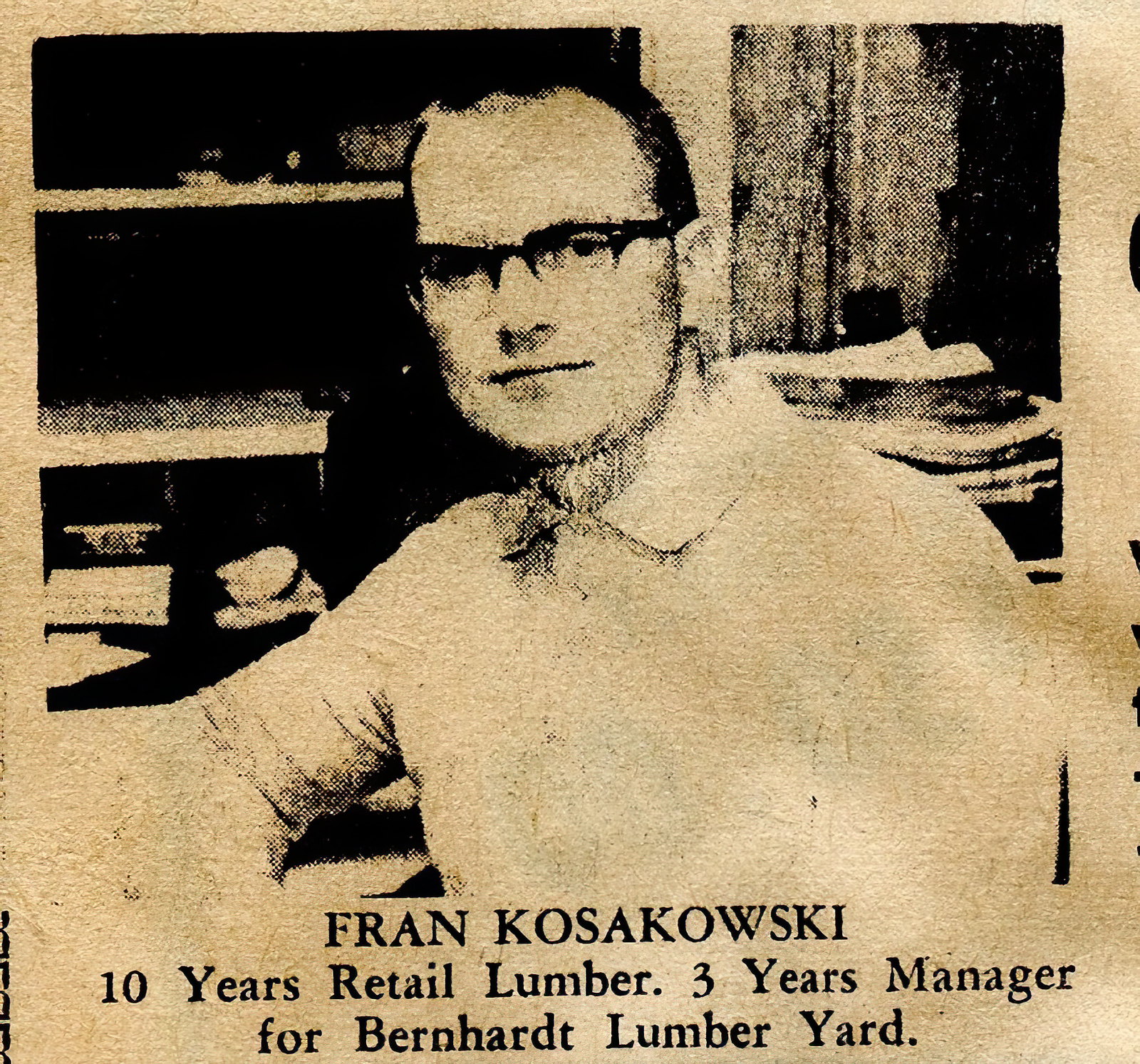The horizontally oriented image, which blends qualities of a photograph and a drawing, features a grainy, almost pointillist style with very fine pencil strokes in black and beige tones. The subject is a man in his mid to late 20s, possessing an air of keen intelligence and self-satisfaction. His short hair and 1940s-50s-era dark-rimmed, pointed-top glasses give him a distinguished look. He sports a slight smile, closed lips, and short sideburns with no additional facial hair. He is dressed in a collared shirt with a sweater over it, and he rests one arm confidently on a desk, where a small desk calendar might be present. Behind him and to his left, there's a set of three shelves, appearing cavernous in the spaces between them, possibly containing books illuminated subtly by side lighting. The background includes a white column and gray curtains, with large stacked papers or art portfolios at the bottom. The aging, sepia-toned image carries a classic newspaper quality, suggesting a mid-20th century origin. The bottom of the image features a tan banner with black Times New Roman lettering, stating "FRAN KOSAKOWSKI," and further specifies "10 years retail lumber, 3 years manager for Bernhardt Lumberyard."